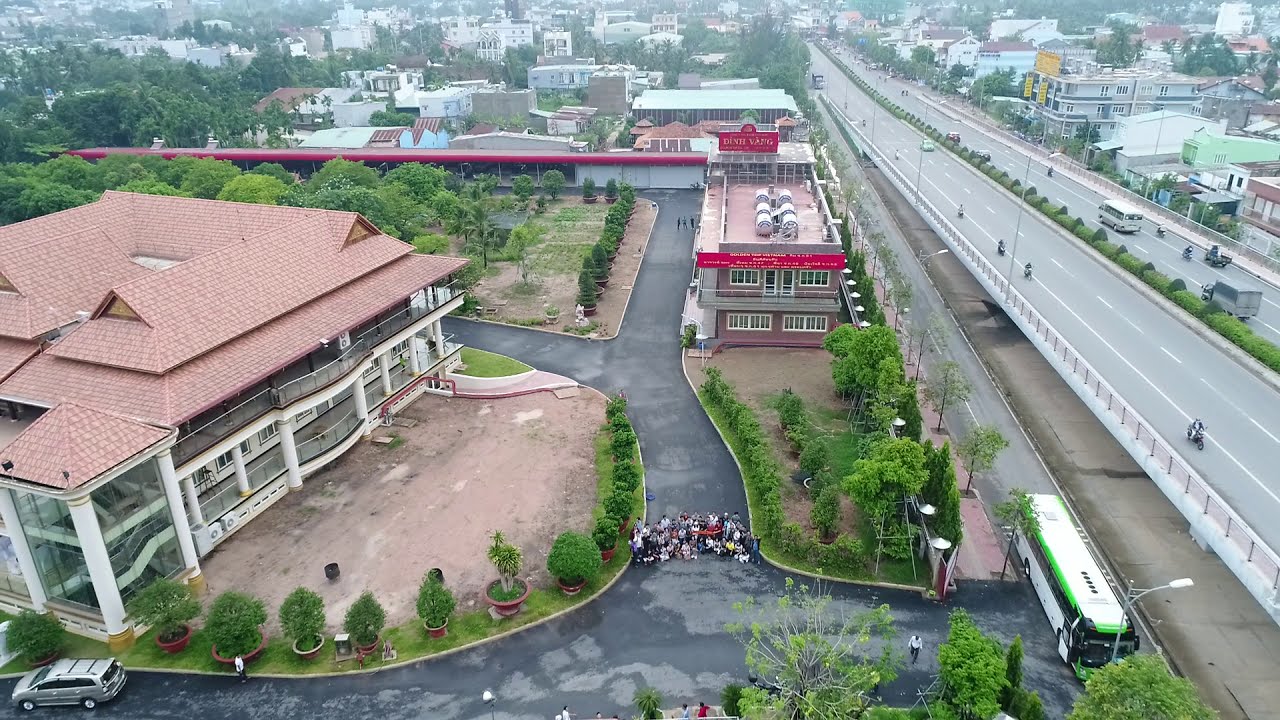This aerial view captures a bustling cityscape with a prominent highway running along the right edge. The highway is divided by bright green shrubbery and features four lanes busy with cars, trucks, and motorcycles traveling in both directions. Flanking the highway on its right side are various types of housing, including apartments and houses, adding to the urban sprawl.

Dominating the left side, the image showcases a mix of residential and perhaps commercial structures. One notable building near the top left corner boasts a red brick roof, white columns, and balconies. This structure is surrounded by a circular driveway and bordered with green potted plants and grass, exuding a grand and well-maintained appearance.

In the midst of this urban layout, there's a roundabout bustling with activity. At the center of the roundabout, a large group of people is gathered, possibly posing for a picture, with others milling around the periphery. Adjacent to the group is a large bus, characterized by a white top, a green streak along the side, and additional black and white coloring, hinting that the group may have arrived on it.

Further adding to the scene's complexity, a two-story building with an orange roof and white columns stands out. It has a glass opening on the bottom left, revealing an interior staircase. Another building nearby is square-shaped with light purple walls, white framed windows, and a rooftop dotted with air conditioners.

Towards the image's far left is a clear area in front of another large structure, trimmed with shrubs and small trees, with a silver minivan parked nearby. Extending into the distance, the cityscape is a mosaic of trees, buildings, and urban life, captured in intricate detail from this elevated vantage point.